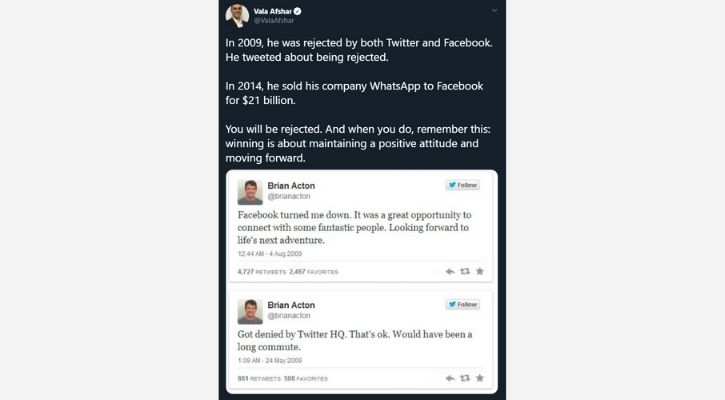**Descriptive Caption:**

A screen capture featuring a tweet by Vala Afshar (@ValaAfshar), identified by a blue verified checkmark beside his username. His profile picture shows a smiling man wearing a white shirt and a black jacket. The tweet recounts an inspiring story about Brian Acton, who was rejected by both Twitter and Facebook in 2009 but later sold his company, WhatsApp, to Facebook for $21 billion in 2014. The tweet encourages maintaining a positive attitude and moving forward after rejection.

Below this tweet is an image showcasing screen captures of two tweets by Brian Acton (@brianacton), each with a "Follow" button, Twitter bird logo, retweet, and favorite icons. The first tweet reads, "Facebook turned me down. It was a great opportunity to connect with some fantastic people. Looking forward to life's next adventure." It is timestamped at 12:44 AM on August 4, 2009, and has 4,727 retweets and 2,467 favorites. The second tweet states, "Got denied by Twitter HQ. That’s okay. Would have been a long commute," timestamped at 1:09 AM on May 24, 2009. The retweet and favorite counts for this tweet are blurry and unclear. Acton’s profile picture shows a brunette-haired man wearing a gray shirt.